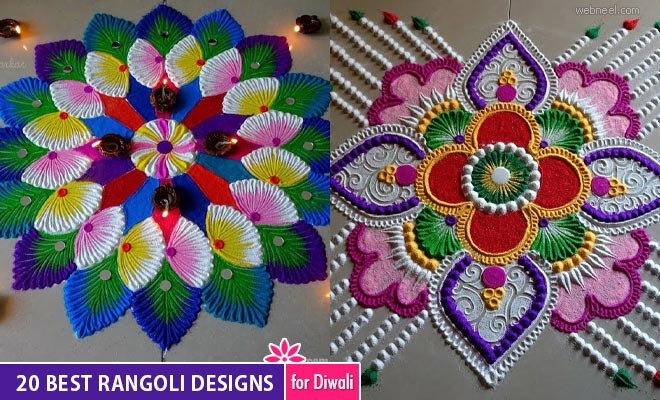The image, likely a screenshot from a video or digital publication, features two distinct and intricately crafted Rangoli designs split into two sections. At the bottom left corner, the text reads "20 Best Rangoli Designs for Diwali," suggesting it originates from an Indian crafting website or book focused on Diwali celebrations.

The left half of the image showcases a vibrant multi-colored Rangoli design, predominantly featuring blue, purple, green, white, pink, yellow, and red hues. This design appears to be illuminated by small black lights, enhancing its intricate patterns and craftsmanship. The surrounding candles add to the festive atmosphere.

On the right, the second Rangoli design is characterized by its detailed artistry, decorated with white, red, yellow, green, purple, and two shades of pink. Unlike the first, it features streaks radiating from each of its four corners, adding a unique dimension to the traditional floral motif. Both designs exemplify the high level of skill and time invested in their creation, embodying the spirit and cultural richness of Diwali.